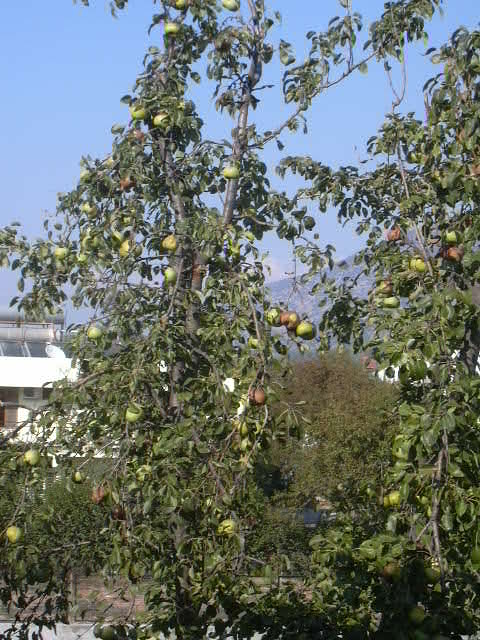The image captures a dense scene dominated by tall, sprawling trees laden with what appear to be green apples. The trees' branches extend in every direction, showcasing a myriad of green leaves interspersed with varying amounts of fruit; some branches carry clusters, while others are sparsely populated. Many of the apples seem underripe, with a hint of red just beginning to appear on a few. In the background, the frame includes a distant mountain ridge tinged with bluish hues, partially obscured by the thick foliage. To the left side of the image, a white house or building peeks through, with its white walls and roof faintly visible, accompanied by what looks like a sidewalk in the lower left corner. The upper portion of the photograph highlights a clear blue sky that provides a serene backdrop to the verdant, fruit-bearing trees.